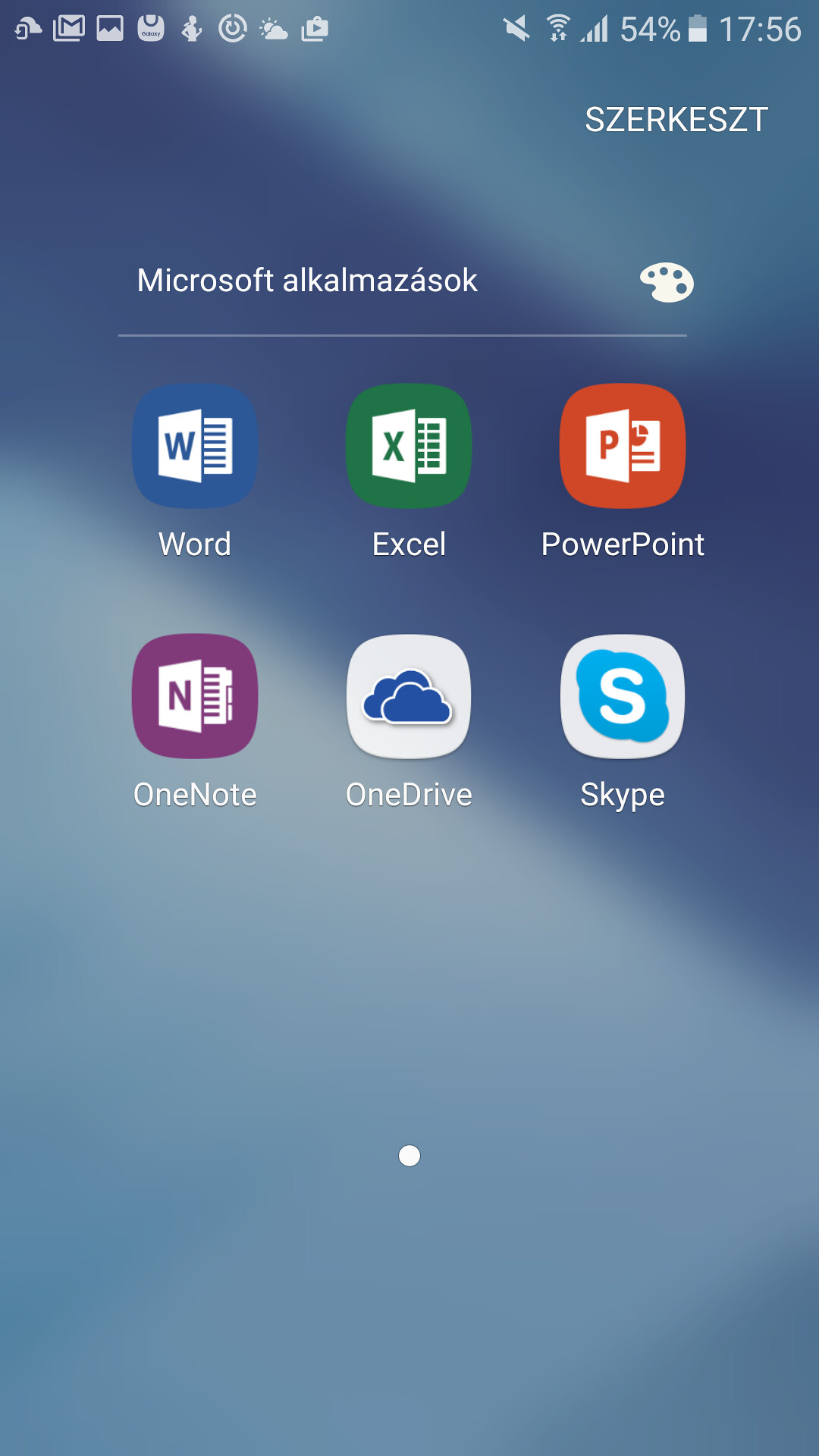**Detailed Descriptive Caption**

The image is a detailed screenshot of an individual's smartphone home screen. The background features an abstract composition of various blue shades: a dark blue band extends from the top left diagonally to the middle right, with lighter blues occupying the bottom and a medium blue at the top right. 

At the top of the screen, there are eight icons aligned in a row, starting with an unidentifiable symbol, followed by a silhouette of a person, a graph icon, and an envelope suggestive of an email app. Another icon appears to represent weather. On the far right, there's a speaker icon with a slash through it, indicating that the sound is muted. Adjacent to it is a Wi-Fi signal icon, accompanied by an illegible label below. A cell signal icon shows full bars, indicating strong reception. The percent symbol followed by “54%” displays the remaining battery life, next to a vertically oriented battery icon. The time reads "1756," which translates to 5:56 PM.

Below these notifications, in all capital letters, are the words "SZERKESZT." Further down, the text "Microsoft Alkalmazások" appears—likely in Hungarian—indicating a section dedicated to Microsoft Office applications. This section is denoted visually by an artist palette icon.

Listed in neat rows are various Microsoft app icons: 
- **Word** (blue background)
- **Excel** (green background)
- **PowerPoint** (red background)

Directly beneath these are:
- **OneNote** (purple background)
- **OneDrive** (blue clouds on a white background)
- **Skype** (stylized white "S" with a blue shape on a white background)

Centered at the bottom third of the screen is a single white dot, which might be for navigation or accessing a home menu. The overall layout suggests a well-organized and functional home screen for productivity tools.